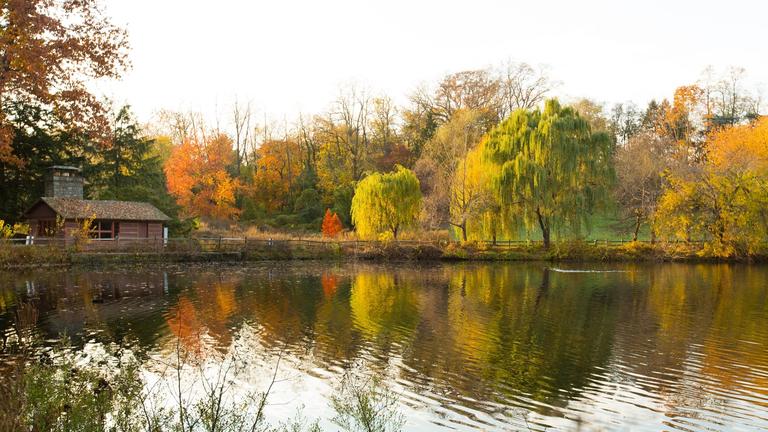The photograph captures a picturesque fall scene set around a small pond or lake, no more than 100 feet across. In the foreground, some plant life and shrubs frame the view. The water is calm but has visible ripples, reflecting the white, hazy sky and a medley of trees adorned in autumn colors—deep greens, vibrant oranges, yellows, and reds—along with some bare branches. On one side of the pond, a dark brown cabin with a large, dark gray stone chimney stands out, its single window overlooking the serene waterbody. Notably, a weeping willow with its long, cascading foliage adds to the scenic beauty. A fence surrounds the lake, enhancing the quaint, tranquil atmosphere of this daytime autumn setting.